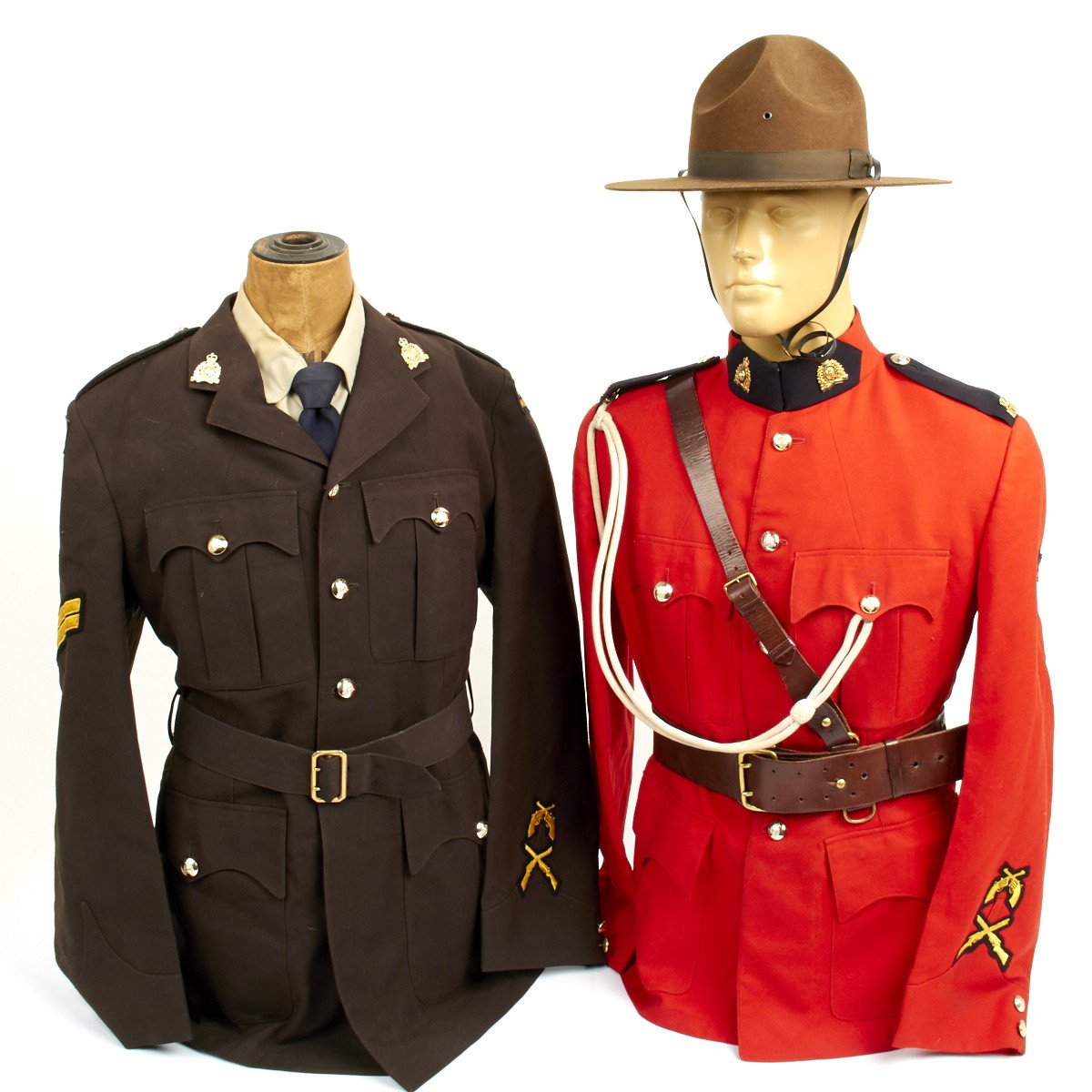This photograph showcases two mannequins dressed in Canadian Royal Mounted Police uniforms. The mannequin on the left, headless, is clad in a brown uniform featuring two chest pockets and silver buttons down the center. A black belt with a silver buckle secures the uniform at the waist, complemented by a beige shirt and a black tie. Notable embellishments include small pins on the epaulets and intricate insignias on the sleeves—specifically, crossed guns. 

In contrast, the mannequin on the right, which has a head, dons the iconic bright red Mountie jacket. This uniform is accessorized with a brown brimmed hat, complete with a chin strap, and is accentuated by a shoulder rope that arcs from the right shoulder to the left breast pocket. Additionally, a brown leather strap runs diagonally from the right shoulder to the belt. The uniform features golden buttons and metallic crossed guns insignias on the sleeves. Both mannequins are adorned with detailed epaulettes and collar pins, enhancing the authenticity and classic appeal of these ceremonial outfits.